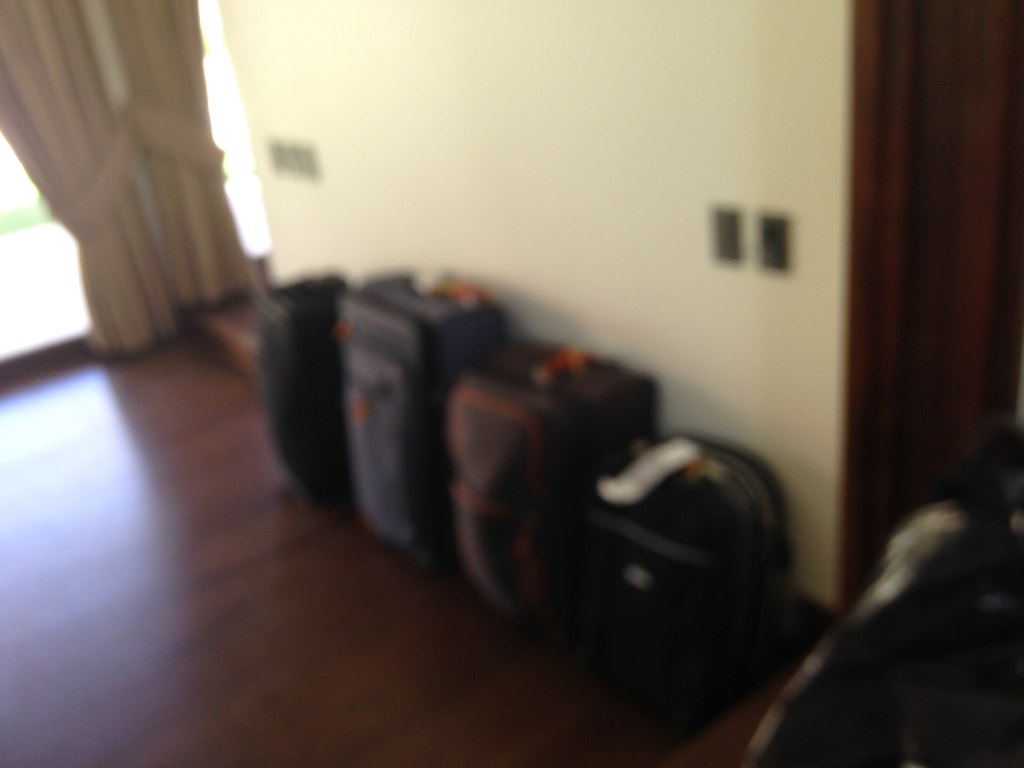In this very blurry photograph taken inside a home, you can make out four pieces of luggage aligned against a beige wall, positioned diagonally across the frame. The quality of the image is poor, making everything appear out of focus. Surrounding the luggage, the scene includes cream-colored and beige curtains, which might look doubled due to a mirror. The luggage itself comprises various colors and sizes: the first one is black, the second one is blue, the third one brown with a lighter brown accent, and the fourth one is black with silver accents. Beside the luggage, you can spot two dark light switches on the wall and a closed dark wooden door on the right-hand side. The luggage is set on a dark hardwood floor, which reflects some light coming through a window to the left. The scene also includes an entryway with a visible window draped with more curtains.